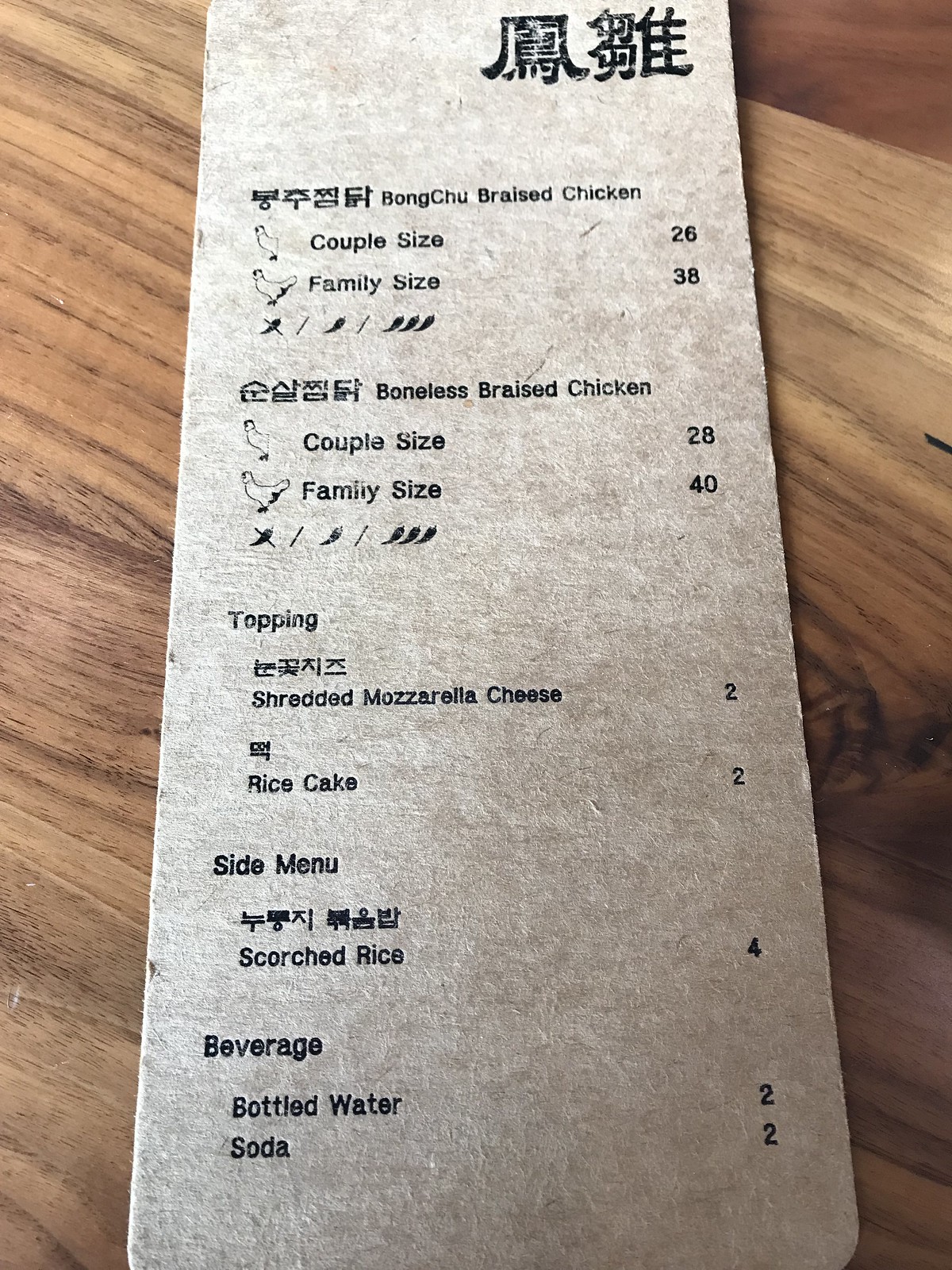The image depicts a menu sticker on a thick paper menu positioned on a brown wooden table. The menu itself is mainly grey with white accents. In the top right corner of the menu, black characters in various languages are visible. Below these, horizontally written characters in a different language can be seen, describing a dish called "bong chu braised chicken," followed by additional text related to heating.

On the left side of the menu, there are illustrations of kitchen tools and beds, presumably representing different preparation or dining options. To the right of these illustrations, there are multiple sections of text:

- "Couple size" is listed first, accompanied by the number "26."
- Further down, "Female size" is mentioned, with the number "38" on the left. These sections are divided by an illustration of a chili plant.
- Below this, "Boneless braised chicken" is listed with two options: "Couple size, 28" and "Family size, 40," also separated by illustrative elements.
- The "Topping" section lists "shredded mozzarella cheese, 2" and "rice cake, 2."
- In the "Side menu" section, "scorched rice" is listed with the price "4."
- Under "Beverage," "bottled water, 2" and "soda, 2" are indicated.

The numbers are aligned on the right side of the image, moving downward, with corresponding text weights on the left side.